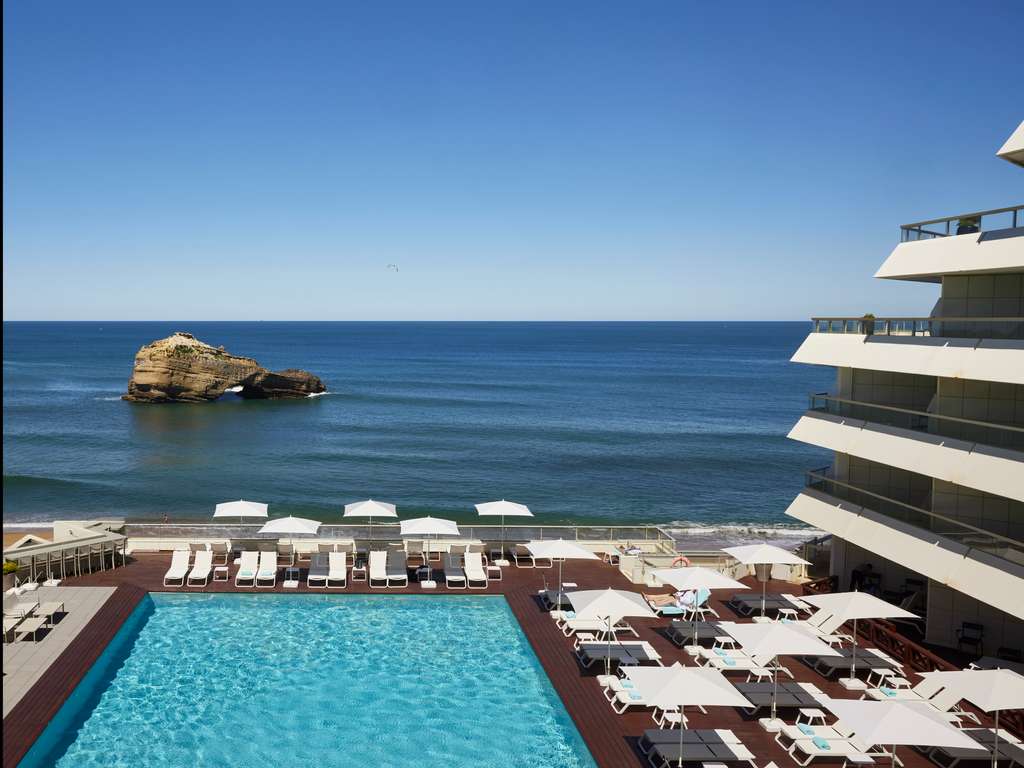This photograph captures a vibrant seaside resort bathed in bright sunshine, making it a perfect vacation destination. The expansive resort features a large, pristine swimming pool, surrounded by numerous poolside chairs and umbrellas where people are basking in the sun and enjoying the warm day. Quite a few guests can be seen swimming in the clear blue pool waters. Adjacent to the pool, on the right side of the image, stands a striking white building with slanted roofs designed to block out the sun's glare, possibly serving as the main resort hotel. This building also features viewing decks that overlook both the pool and the sea.

The scene transitions smoothly to a sandy beach near the ocean, dotted with people walking along the shore and a few tents and umbrellas set up for shade. The ocean itself is a mesmerizing, blazingly blue expanse with waves gently lapping against the shoreline. In the distant background, a natural rock formation juts out of the water, adding a dramatic element to the serene seascape. The sky above is a clear, cloudless blue, completing the picturesque and inviting coastal setting.